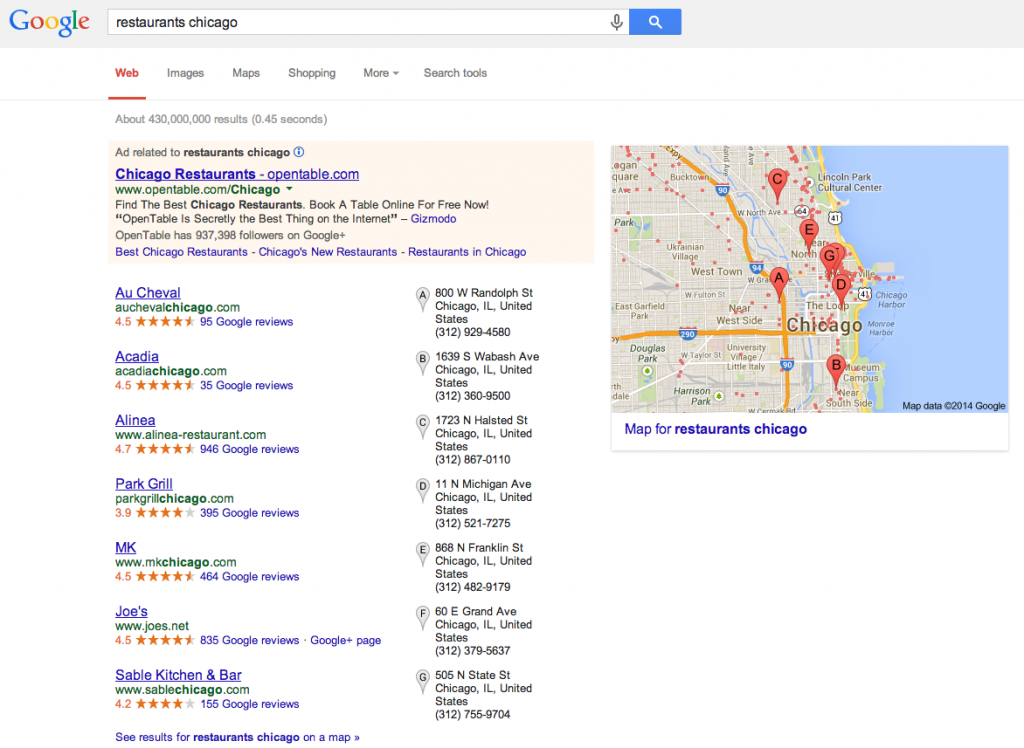This image showcases a Google search results page for "restaurants Chicago." At the top left, the familiar Google logo is visible, with the search query displayed prominently in the search bar. The left side of the page lists detailed information about seven restaurants, beginning with "Au Cheval." Each restaurant listing includes the name, website link, star rating, Google reviews, address, and phone number. Following "Au Cheval," the other restaurants listed are "Acadia," "Alinea," "Park Grill," "MK," "Joe's," and "Sable Kitchen and Bar."

On the right side of the page, a map of a portion of Chicago is displayed. In the bottom right corner of the map, “Map data ©2014 Google” is noted. The map shows Lake Michigan on the right and various sections of Chicago on the left. The map features numerous small dots representing different places of interest, although most are unlabeled. However, several red-orange pins with letters from A to G correspond to the listed restaurants. Notable areas such as Ukrainian Village, West Town, Near West Side, Chicago Harbor, and Harrison Park are labeled. These labeled areas help users visually locate each restaurant, with the "A" pin on the map corresponding to "Au Cheval" and so forth through "G."

The overall composition provides a comprehensive visual and textual representation of some of Chicago's dining options, complete with ratings, contact information, and geographic context.